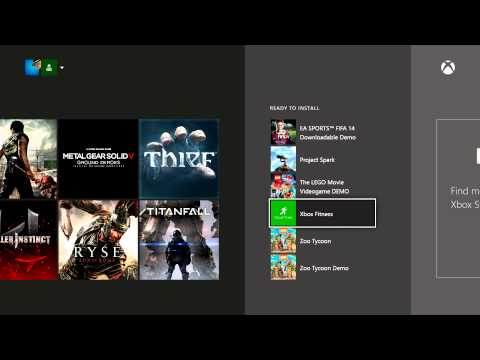The image is a screenshot from the Xbox app, although it is quite blurry. Despite the lack of clarity, the app interface shows various game thumbnails, likely serving as cover art for the titles. On the left side of the image, a few discernible game covers include "Metal Gear Solid V," "Thief," "Killer Instinct," "Ryse: Son of Rome" (spelled R-Y-S-E), and "Titanfall." These appear to be listed under the section of installed games. 

Meanwhile, in the center-right section of the image, a panel labeled "Ready to Install" displays several games that are available for installation. This list includes "EA Sports FIFA 14," "Zoo Tycoon," "The Lego Movie Video Game," "Project Spark," and "Xbox Fitness." Notably, "Xbox Fitness" is highlighted, implying that the user might be preparing to install this particular game. Overall, the image suggests a typical layout where installed games are shown on one side, and games ready for installation are shown on the other.